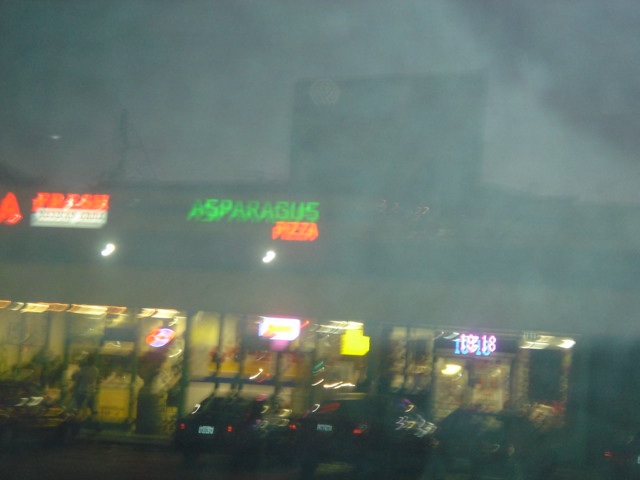Despite the blurry quality, this image vividly portrays a fog or smog-shrouded storefront area, adding an eerie ambiance. The focal point is a brightly lit store named "Asparagus Pizza." The signage features the word "ASPARAGUS" in striking red, capital letters, highlighted in green, while "Pizza" is highlighted in red. The store is well-illuminated, signaling its lively business. Adjacent to Asparagus Pizza, on the left, is another bustling establishment, visible through the lit windows with customers inside. In front of these businesses, several cars are parked, emphasizing the area's active nightlife despite the foggy conditions.